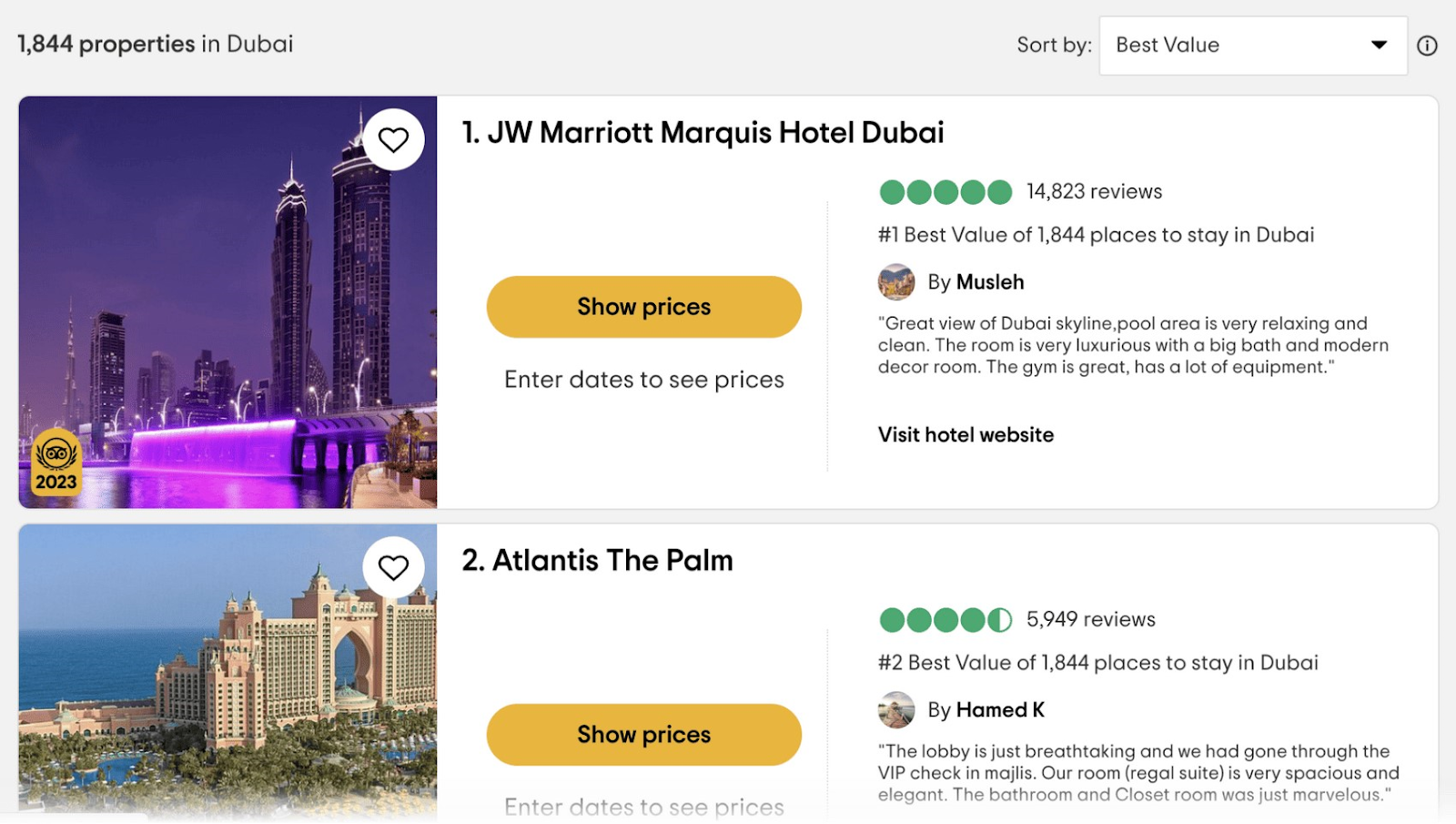A screenshot of a tablet displays search results for 1,844 properties in Dubai, sorted by "Best Value" on a drop-down menu located on the right side.

At the top of the results, **JW Marriott Marquis Hotel Dubai** is listed as the number one best value place to stay in Dubai. It boasts 14,823 reviews and holds a five-star rating, visually represented by green circles. An accompanying review by Mosleh praises the hotel for its great view of the Dubai skyline, a relaxing and clean pool area, and luxurious rooms adorned with modern décor, including a spacious bath. The hotel's gym is also commended for its extensive equipment. A bold black link below the review directs users to the hotel's website. A nighttime photo of the hotel is displayed on the left, featuring a "2023" award symbol. Users can favorite the listing by clicking a heart icon or check room prices through a yellow “Show Prices” button, which opens a date entry field.

The second listing is for **Atlantis, The Palm**, ranked as the second best value hotel among the 1,844 properties. This hotel has garnered 5,949 reviews and holds a four and a half-star rating. A review by Hamid K is displayed below the listing. Similar to the first result, it includes a photo of the Atlantis on the left, along with identical buttons for favoriting the listing and checking room prices.